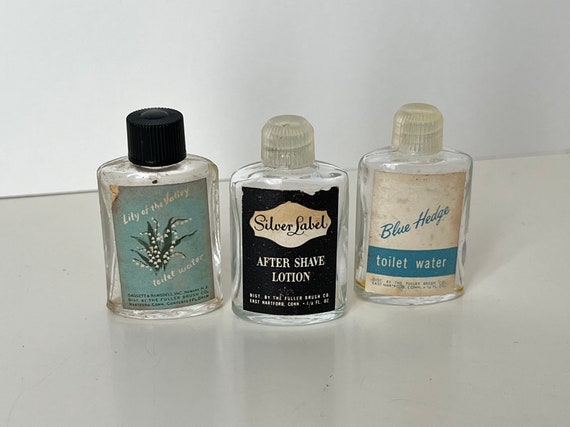This amateur photo showcases three vintage, travel-sized vials of toiletries, displayed against a white backdrop with a white and grey bottom. Each vial, holding approximately one ounce of liquid, evokes the nostalgic charm of hotel amenities from the 1950s or 60s, evidenced by their old, worn labels. 

On the left stands a vial with an aqua-colored label featuring a botanical illustration and marked "Lily of the Valley Toilet Water," capped with a distinct black top. The centerpiece is a black bottle with a silver label reading "Silver Label Aftershave Lotion," its text strikingly clear against the dark background. The rightmost vial, similar in shape and size to the middle one, boasts a white label with a blue stripe at the bottom inscribed "Blue Hedge Toilet Water" in blue font, and it shares the same clear cap as the aftershave lotion. This trio of bottles, set against a simplistic and neutral backdrop, captures the essence of vintage grooming elegance.